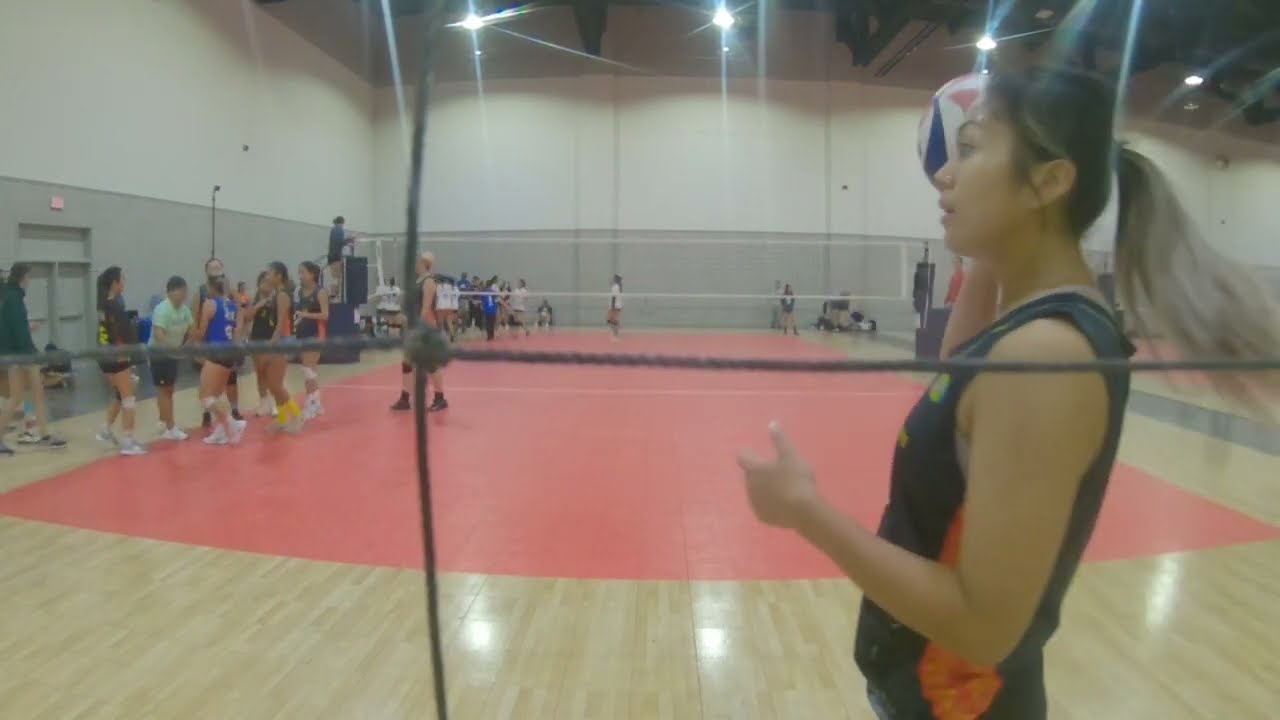The photograph captures an indoor volleyball court with a wooden floor, which might also serve as a basketball court, given the pinkish-orange lines on the floor. The image appears to be taken through the net, as faint strings of netting obscure parts of the scene. Dominating the right side of the frame is a female volleyball player in a sleeveless black jersey with an orange stripe and a small green button on the chest. She has olive skin, dark hair tied in a ponytail, and holds a volleyball with red, white, and blue triangular sections in her right hand, poised to serve. Her left hand is extended across her body. On the left side, a group of around six or seven players, all wearing similar outfits, is clustered around a person in a green shirt. There's also someone who seems to be the judge standing beside the net in black. The ambient scene captures the pre-game anticipation and camaraderie among the players, emphasizing the lively and focused atmosphere of the gymnasium.